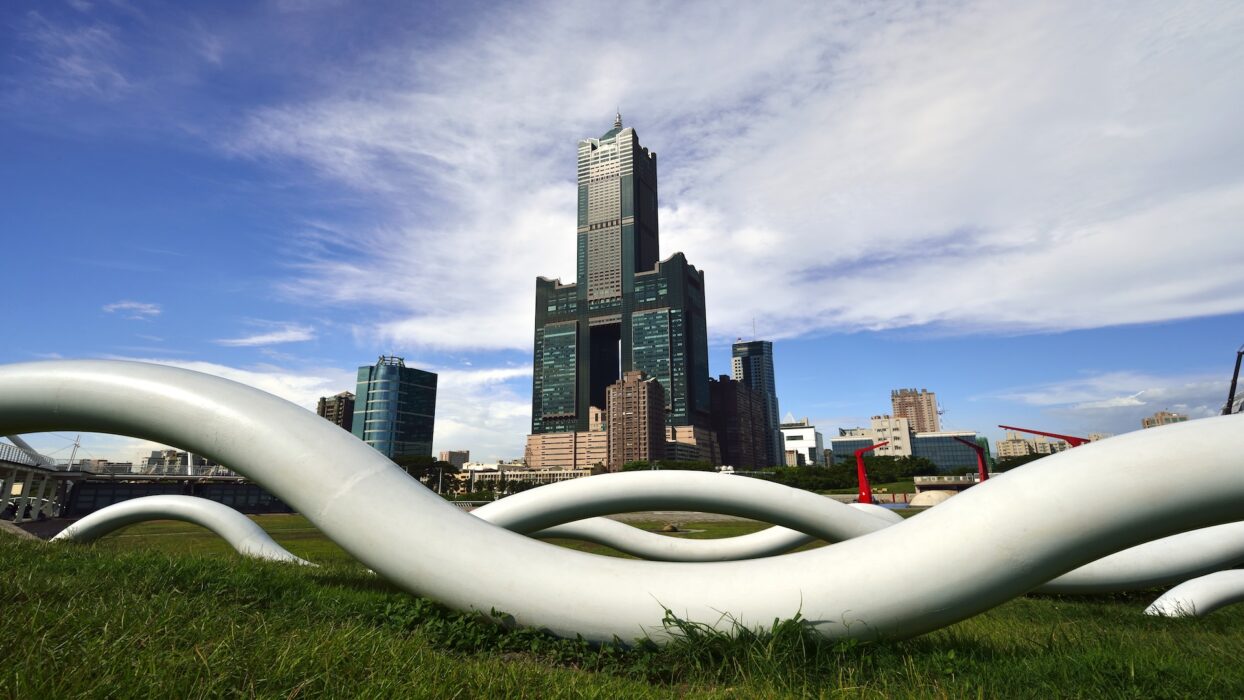The photograph captures a large white wavy tube-like sculpture set in a grassy field. The sculpture, composed of reflective tube structures, undulates up and down, creating spaces beneath it that one could walk under. In the foreground, we see the base of the first tube, with subsequent sections forming two humps before disappearing into the grass. Surrounding the sculpture is a fence adorned with red posts. In the background, a mid-sized downtown skyline features prominently, dominated by a tall turquoise skyscraper topped with a pyramid shape, accompanied by smaller white and tan buildings. The blue sky above is partly covered with white clouds, adding depth to the city's silhouette.